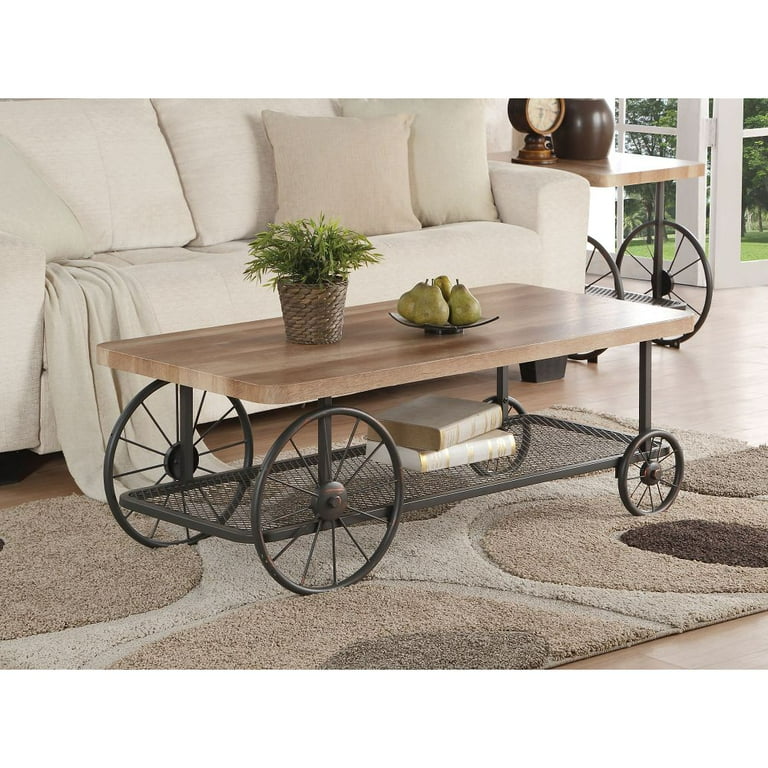The photograph, evocative of a home magazine or Realtor ad, captures a stylishly decorated living room. Dominating the foreground, a white three-seater sofa, partially cropped, is adorned with two pillows and a cozy blanket. In front of the sofa stands a unique coffee table with a warm wooden top and a metal grate shelf beneath. The table showcases a small plant in a brown wicker planter and a bowl of pears. Below, on the metal shelf, lie two books. The table's design is accentuated by its unconventional wagon-like wheels, with the left pair notably larger than the right. 

Beside the sofa, a matching side table, also equipped with similar distinctive wheels, holds a clock. Both tables rest on a gray and brown rug featuring an abstract pattern of large circles. The room's flooring is light-colored hardwood, adding to the space's airy yet cozy feel. In the background, an open door and windows with white frames allow natural light to spill into the room, further enhancing its welcoming ambiance.